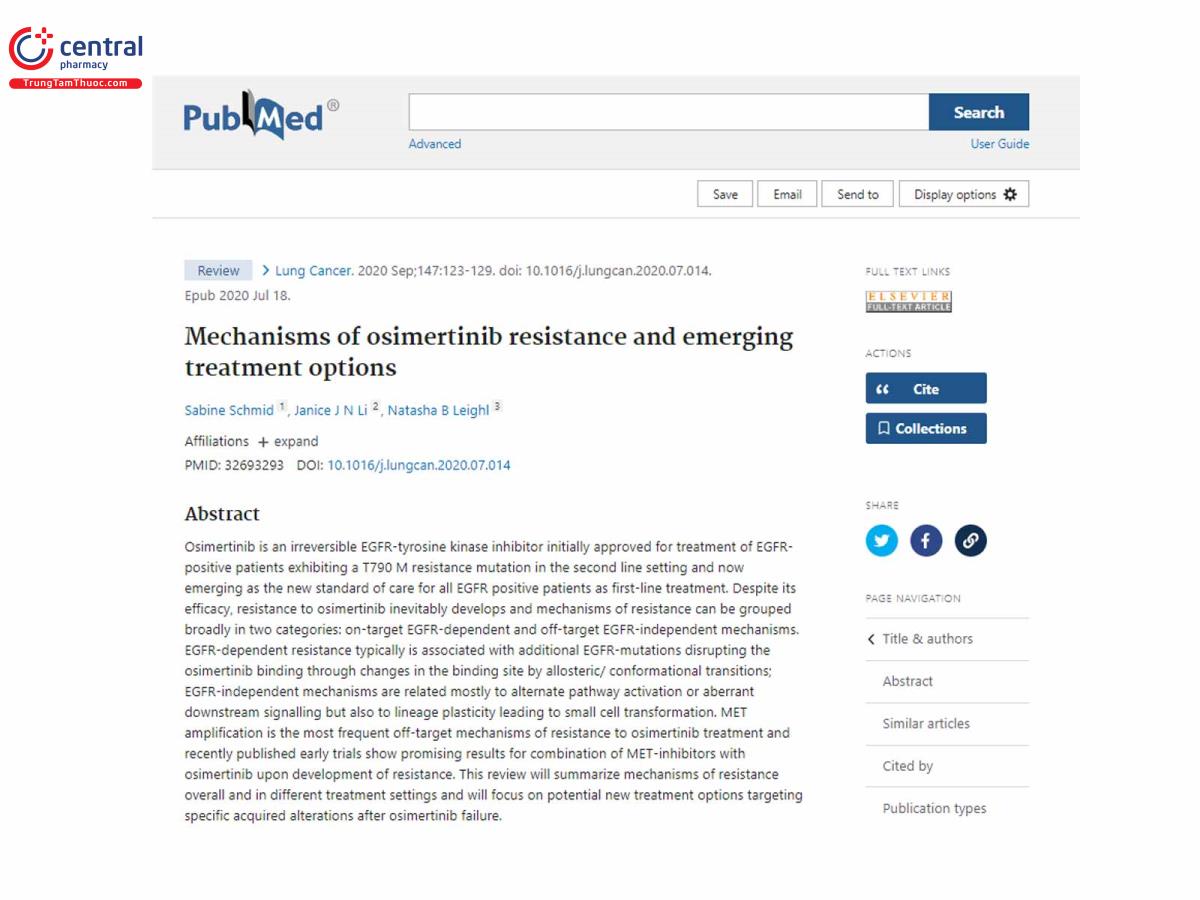On a clean white background, the interface of Central Pharmacy's PubMed search page is displayed, showcasing a variety of tools and sections for detailed medical searches. At the top, a search bar is prominently featured, with the text "Advanced" in blue directly beneath it. To the right of the search bar, a blue rectangular button labeled "Search" in white text is visible.

Below the search bar, several options are arranged, including "User Guide" in blue, "Save," "Email," "Send to," and "Display Options," accompanied by a settings icon. The page displays a search result for "Review Lung Cancer, September 2020" with the citation SEP 147:123-123. 

Beneath this, there are links to "Full Text Links" and "Actions." Two additional blue rectangular tabs are visible, marked "Site" and "Collections" respectively. The highlighted abstract titled "Mechanisms of Osimertinib Resistance and Emerging Treatment Options" provides an overview. It states that Osimertinib, an irreversible EGFR tyrosine kinase inhibitor, was initially approved for treating EGFR-positive patients with a T790M resistance mutation in the second lung cancer setting, and its emerging applications in treatment.